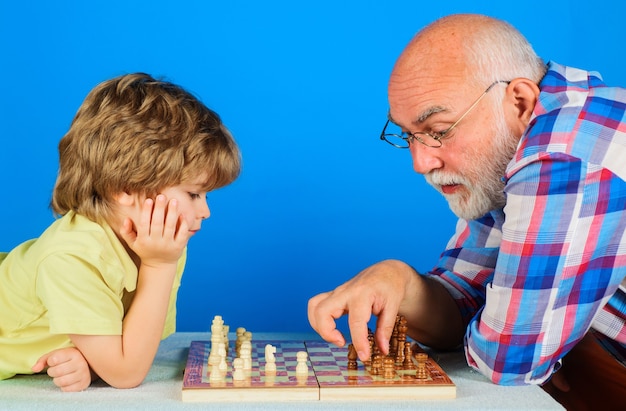The image features a meticulously staged scene of a small child and an elderly man engrossed in a game of chess, set against a studio backdrop that transitions from lighter to darker shades of blue. The chessboard is centrally positioned at the bottom of the image atop a table. The young boy, who appears to be around five years old, is positioned on the left side. He has shaggy light brown hair and is wearing a yellow t-shirt, resting his elbow on the table with his right hand on his cheek as he contemplates his next move. The older gentleman, approximately in his late sixties to seventies, is on the right side of the image. He is balding with gray hair and a beard, and wears glasses along with a plaid shirt featuring shades of red, blue, and white. His hand is poised over a dark wooden chess piece, indicating he’s in the midst of making a move. The chess pieces on the young boy's side are white, while those in front of the older man are a deep brown, wooden color. The setting and their engagement in the game suggest a thoughtful and lighthearted interaction between two generations.